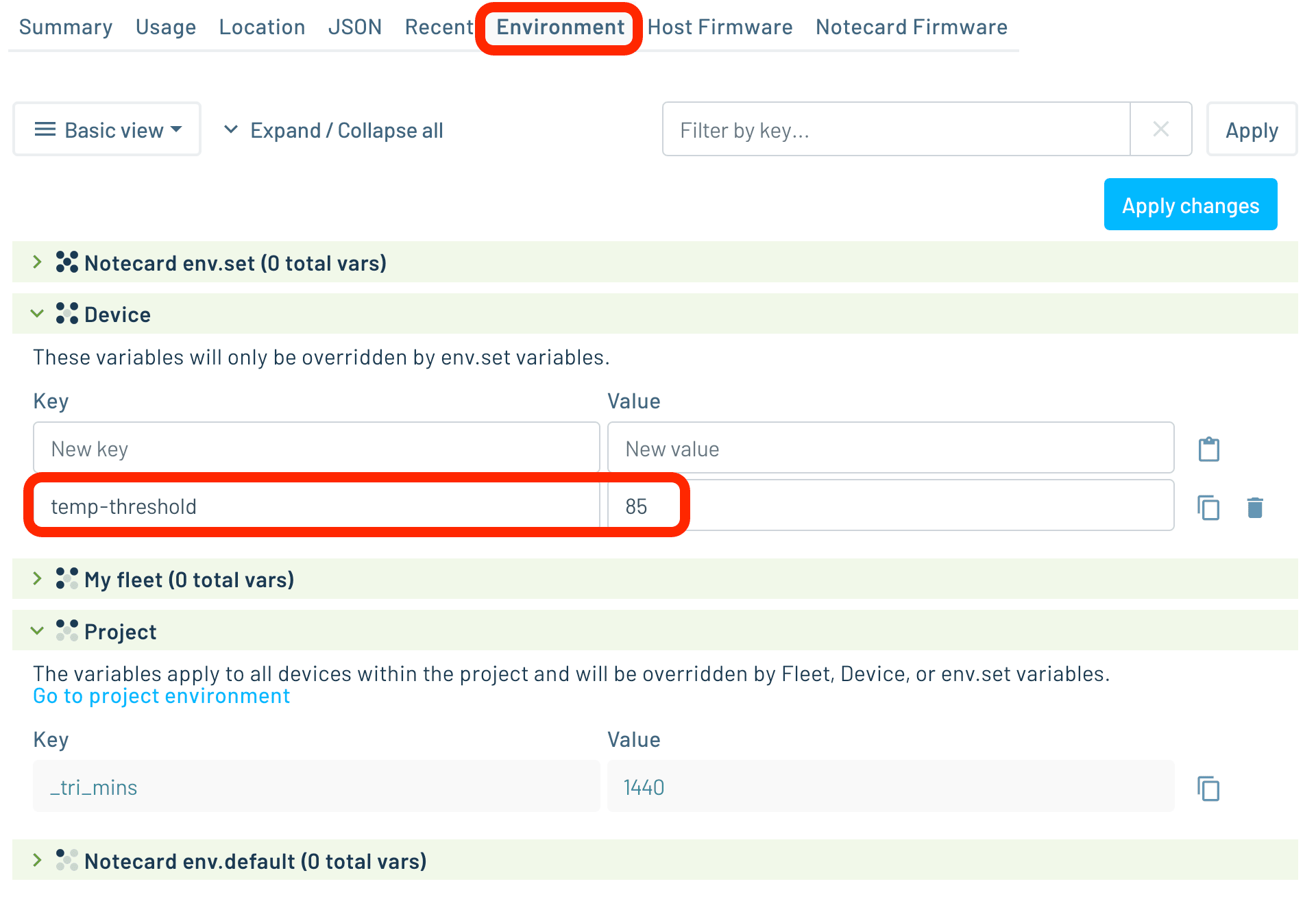This screenshot from a website depicts a form that predominantly features black text on a white background, interspersed with green rectangles for emphasis. The top navigation bar includes tabs titled "Summary," "Usage," "Location," "JSON," "Recents," and "Environment," with the "Environment" tab highlighted by a red rectangular outline. This outline also encloses "Host Firmware" and "Notecard Firmware."

Beneath this, the form allows the user to toggle between "Basic View" and a dropdown menu option for "Expand/Collapse All." A search filter labeled "Filter by key" is accompanied by an "Apply" button. On the right-hand side, a blue button labeled "Apply Changes" stands out.

Within the form, two green rectangles are present. The first reads, "Notecard, env, set, zero total vars," and the second is labeled "Device." Both have associated dropdown menus on the left. Under these titles, it is noted that the variables will only be overwritten by environment-set variables. Specifically, a key field reads "Temp Threshold," with a corresponding new value entered as "85."

A red rectangle superimposes these fields, encompassing them within its borders. Further down, another green rectangle titled "My Fleet, zero total vars," and an additional one labeled "Project," are shown. It's indicated that these variables apply to all devices within the project and will be overwritten by fleet, device, or environment-set variables. Blue text directs users to "Go to project environment."

Finally, another key field displays "TRI mins," with a value entry of "1440" beside a copy and paste icon, followed by another green rectangle labeled "Notecard, env, default, zero total vars."